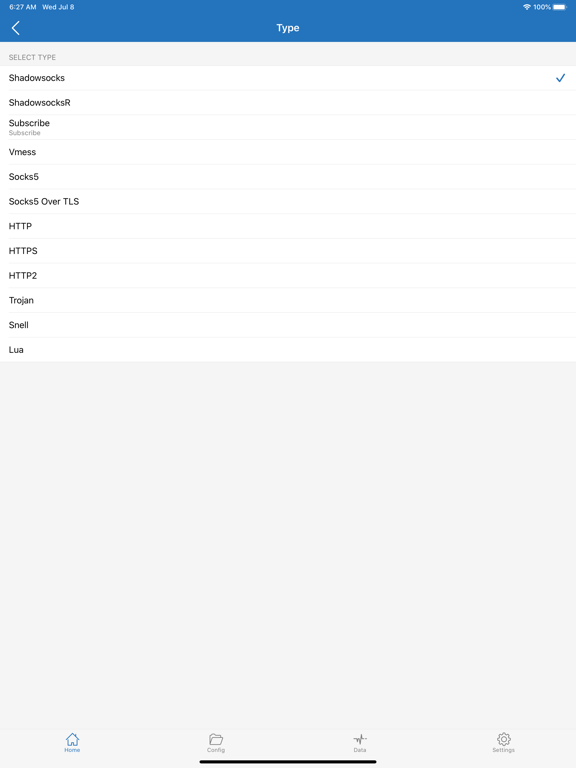This image is a large screenshot that appears to capture the display of a computer or possibly a cell phone screen. At the top of the screen, there is a blue banner stretching across the full width. This banner contains various pieces of information: on the left side, it displays the time "6:27 a.m." and the date "Wednesday, July 8th" in abbreviated form. In the middle of the banner, there is the word "Type". On the right side, the banner shows a Wi-Fi signal icon, a "100%" indication, and a battery life symbol.

Below this banner, the main section of the screen appears, titled "Select Type", offering a list of options in mostly black text. The options are as follows: 
1. ShadowSocks
2. ShadowSocksR
3. Subscribe
4. Another "Subscribe" option in lighter gray
5. VMess
6. Socks5
7. Socks5 over TLS
8. HTTP
9. HTTPS
10. HTTP/2
11. Trojan
12. Snell
13. Lua

At the bottom of the screenshot, there are four navigation buttons labeled "Home", "Config", "Data", and "Settings".